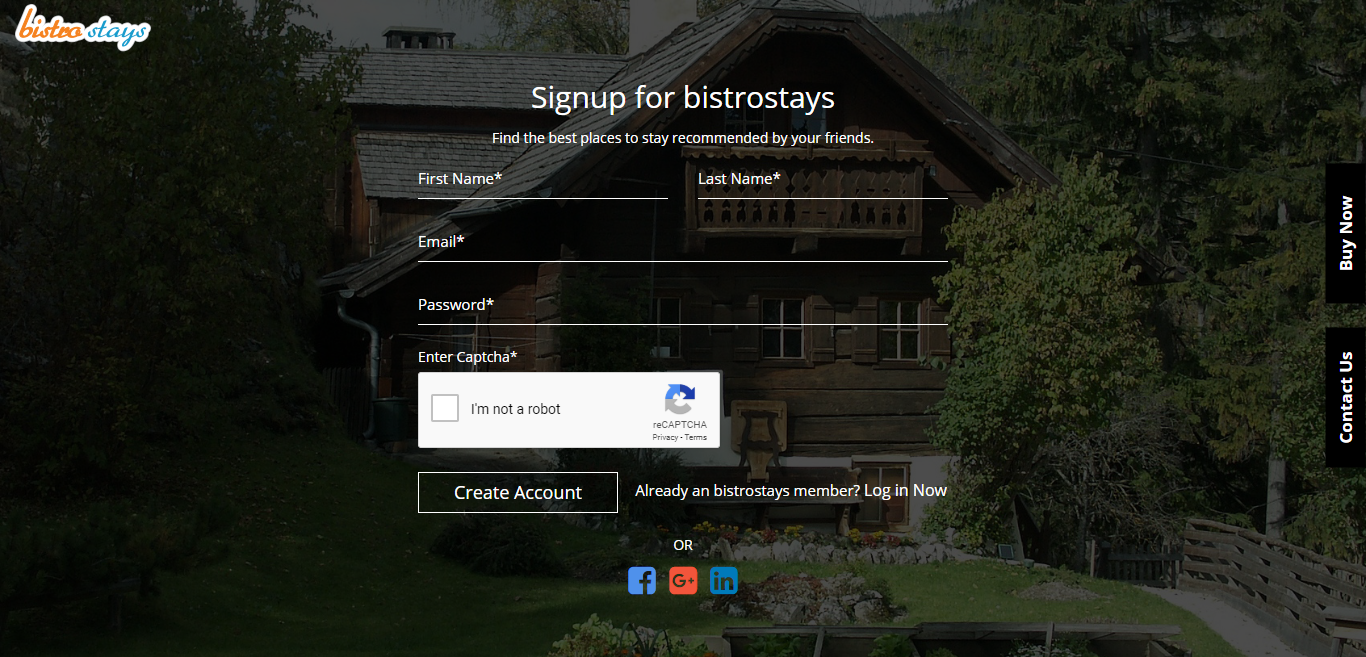The screenshot depicts a website page in landscape orientation, featuring a dark and professional photograph as the background. On the left side of the image, the scene is largely obscured by darkness, but you can discern the faint outlines of trees. The right side is slightly brighter, allowing for clearer visibility of the trees and revealing a somewhat illuminated, ornate, three-story cabin nestled among them.

At the forefront, there is a text overlay that reads: "Sign up for Bistro Stays - Find the best places to stay recommended by your friends." The word "Bistro" is emphasized.

Below this message is a registration form with fields for "First Name," "Last Name," "Email," and "Password." Additionally, there is a CAPTCHA for verifying that the user is not a robot. At the bottom left of the form, a button labeled "Create Account" is displayed, while to the right, a prompt reads: "Already an Bistro Stays member? Log in now," with "now" in bold to indicate it is a clickable link.

Further down, the page offers alternative sign-in options via social media platforms, listed as Facebook, Google+, and LinkedIn. Along the right edge of the image, two prominent black buttons are vertically aligned, stating "Contact Us" and "Buy Now" respectively. The overall composition combines functionality with visually appealing elements to encourage user engagement.